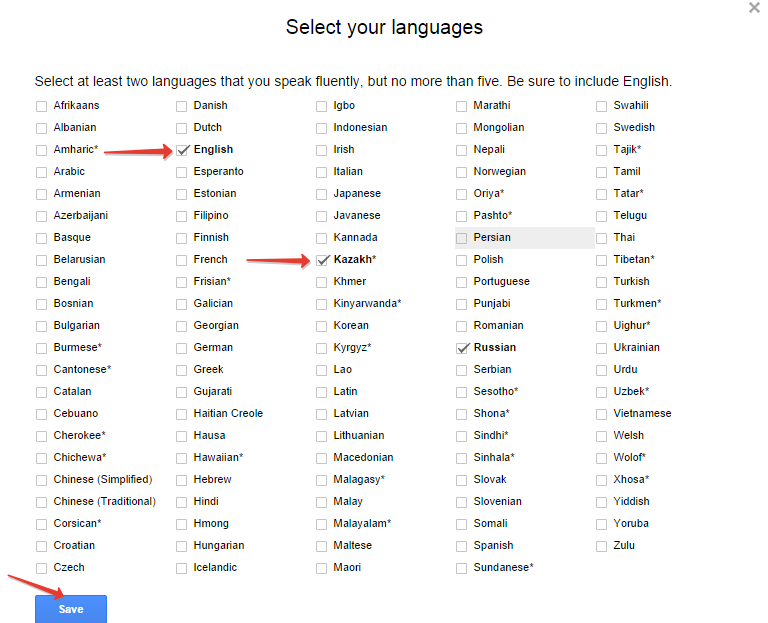In the image, a user is in the process of selecting languages for a particular application interface. The user has chosen English and Kazakh as their primary languages, as indicated by red arrows pointing at both languages along with a star next to Kazakh. Additionally, the blue "Save" button to confirm the selection is prominently displayed. Russian is also checked as a selected language, although it lacks the guiding red arrow present on English and Kazakh. Persian appears in the selection list but is only highlighted in gray without a checkmark, indicating it has not been chosen.